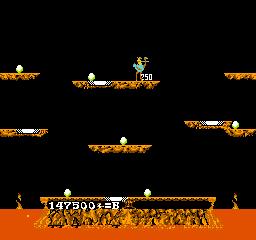This image showcases a classic 8-bit video game scene reminiscent of retro Nintendo or Sega aesthetics. The bottom portion of the screen is dominated by a landscape resembling red volcanic ash, which transitions into a stone base outlined with a black border. Inscribed within the black edging is a score display. Erupting from the volcanic terrain are animated flames that add a dynamic visual element.

Central to the scene are two vertical pillars with pointed tops, featuring a textured pattern. Atop the tallest pillar stands a blue, long-legged bird, seemingly supporting a rider. The number "250" is displayed adjacent to the bird, indicating either a score or a level marker.

Accompanying these main structures are several floating pillars along the sides, some of which bear eggs, contributing to the game's intricate environment. The entire scene is set against a deep black background, highlighting the vivid colors and pixelated charm of the game's graphics.